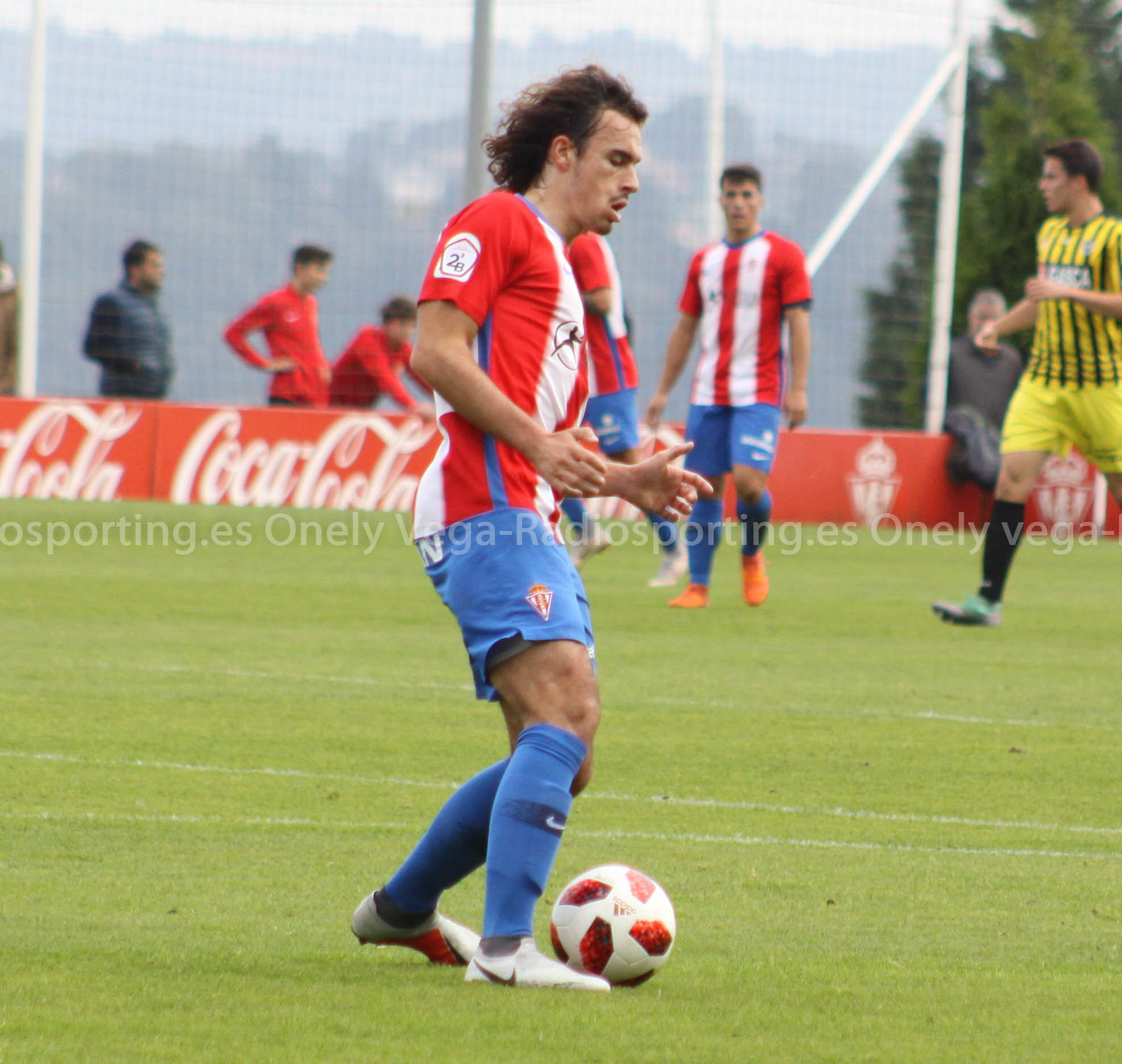In this vibrant and well-detailed image of an ongoing outdoor soccer match, the focal point is a player dribbling a white soccer ball adorned with red markings. This player, standing centrally, is donning a red and white striped jersey, blue shorts, knee-high blue socks, and white cleats. His dark, curly hair flows as he maneuvers the ball skillfully on a lush, green field. 

In the background, to the left, a teammate stands upright, dressed similarly in a red and white striped top, blue shorts, and different colored shoes. On the right edge of the frame, a player from the opposing team enters the scene, distinguishable by his yellow shirt with black vertical stripes, yellow shorts, and black socks. 

The backdrop of this match features a prominent red banner emblazoned with the 'Coca-Cola' logo in white, signaling the popular beverage brand as a sponsor. Additionally, large nets surround the field to prevent the ball from exiting the play area, ensuring the game continues smoothly and safely.